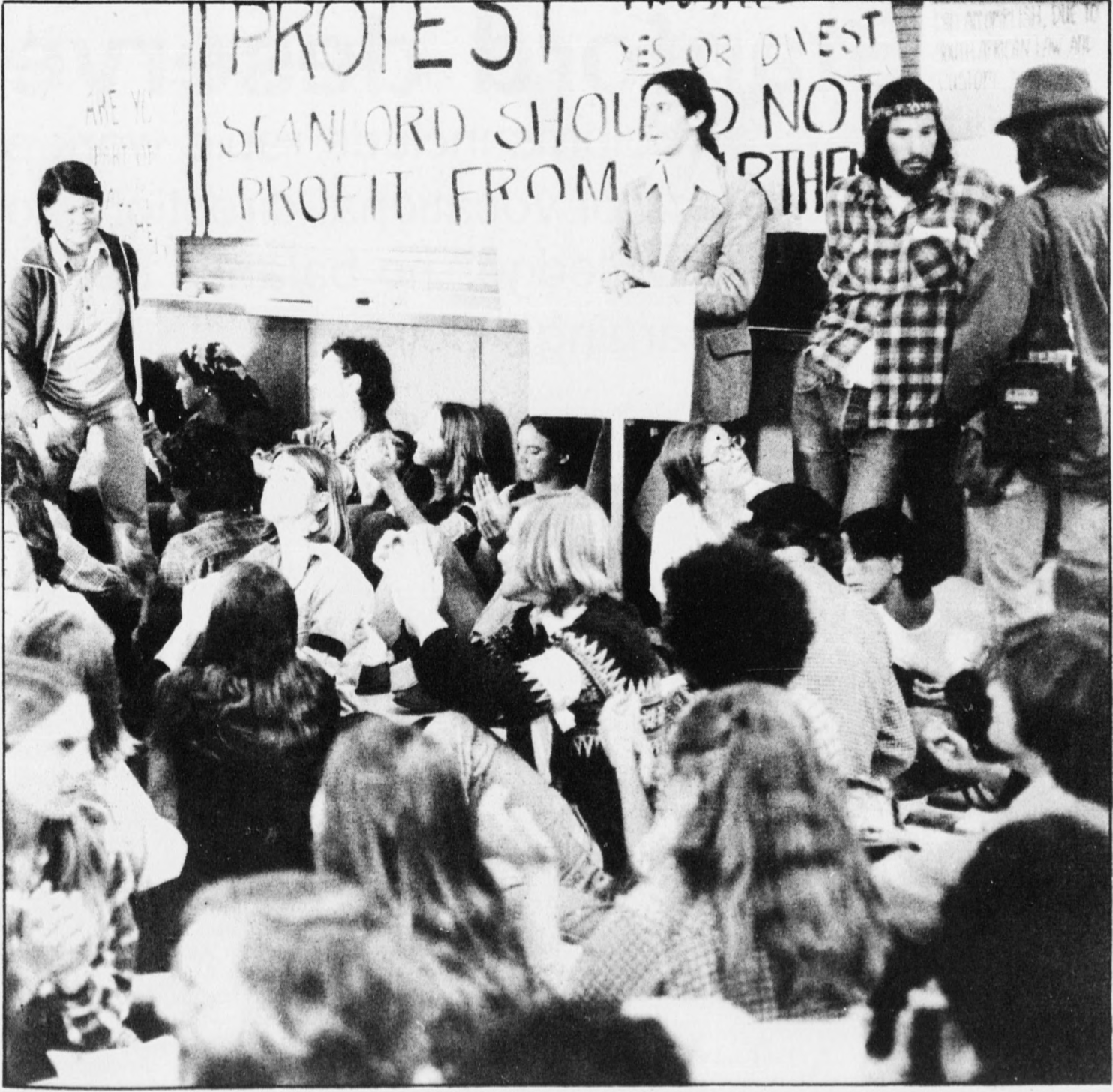This black-and-white photograph captures a 1969 Vietnam War protest at Stanford University. In the foreground, a diverse group of young adults—many with long hair, headbands, and facial hair typical of the hippie generation—are engaging in conversations. Central to the image, a female protester in a blazer holds up a sign, while beside her, two young men talk animatedly. The background is dominated by a large, partially obscured banner reading "Protest: Stanford Should Not Profit From [unreadable text]." The scene is bustling with activity, as students sit and stand on various objects, voicing their opposition and advocating for divestment. The high contrast of the black-and-white format lends a vintage aura to the charged atmosphere of this explosive demonstration.